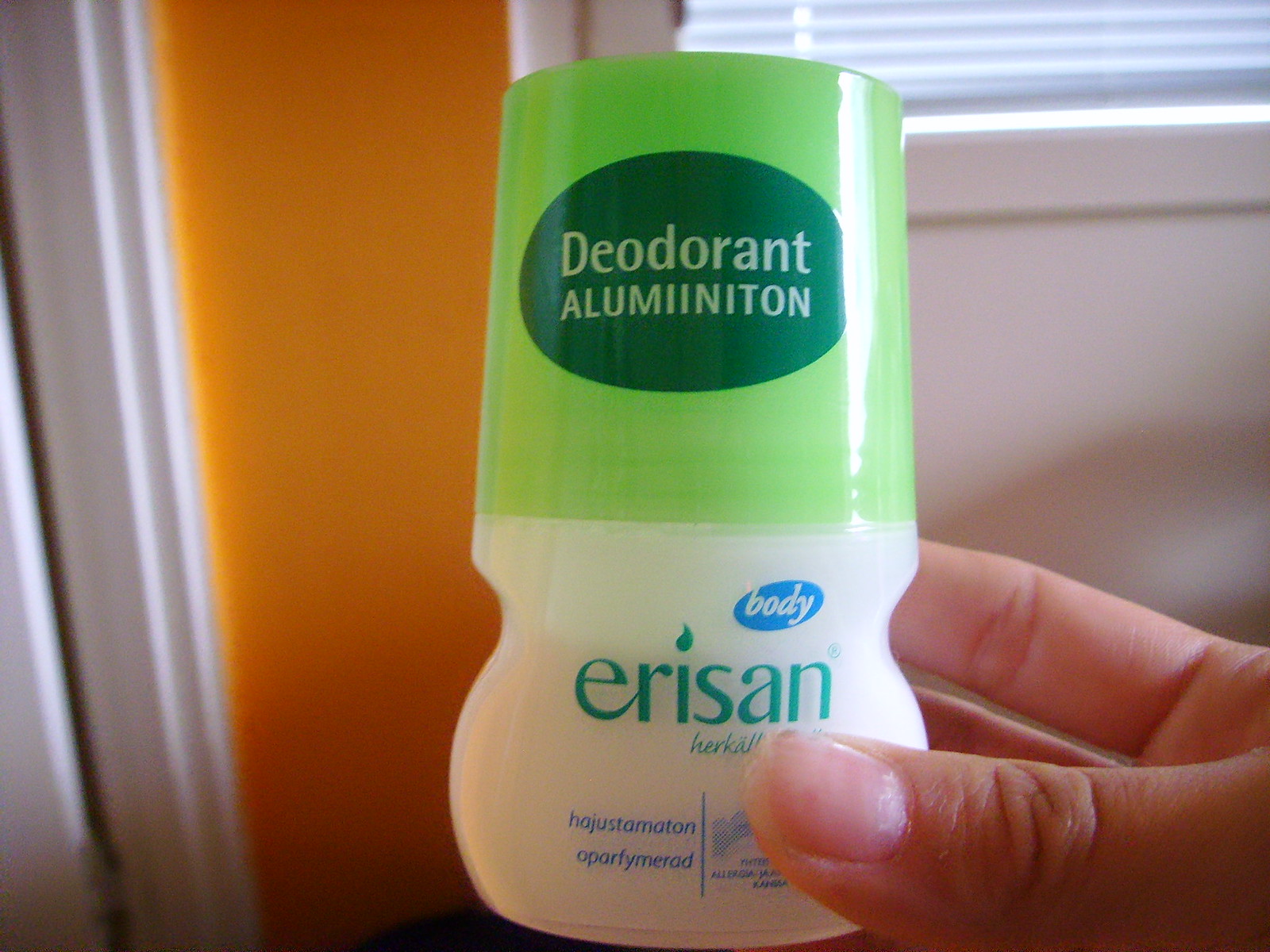A person with fairly light skin is holding a deodorant bottle in their hand, extended from the lower right side of the photograph. Their thumb is visible on the front and two fingers wrap around the back of the bottle. The deodorant features a lime green cap adorned with a forest green horizontal oval sticker. On the sticker, "deodorant illumination" is printed in white sans serif font. The white deodorant container is ergonomically designed with a slight curvature. It prominently displays the brand name "ERISAN" in green letters, and above it, a blue horizontal oval with the word "body" in white. Further down the label, additional text reads "HAJUSTAMATON" and "OPARFYMERAAD." The background reveals part of a door frame and an orange wall on the far left, while behind the hand, there is a white wall with a section of a window featuring mini blinds visible at the top.